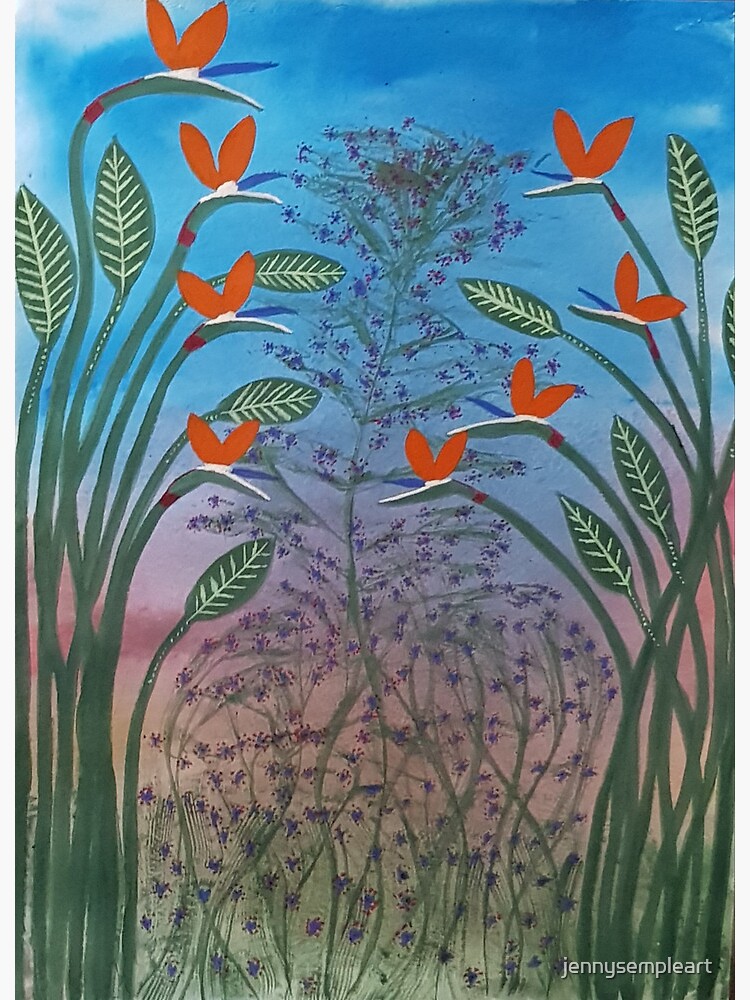The painting features a vibrant depiction of plant life set against a gradient sky. Central to the composition is a vine-like plant with delicate, tiny purple flowers, reminiscent of lavender. This plant is flanked by taller greenery on the left and right, some adorned with orange-tinted leaves and butterflies. The leaves display intricate white veins. The sky transitions from a bright blue at the top through light lavender, maroon, and ultimately to a reddish-yellow hue near the horizon, evoking a sunset ambiance. The artwork is signed "Jenny's Simple Art" in the bottom right corner. Overall, the painting combines a rich palette of colors including orange, reddish-brown, light green, sky blue, purplish violet, maroon, and reddish-yellow, bringing the scene to life with a sense of warmth and tranquility.